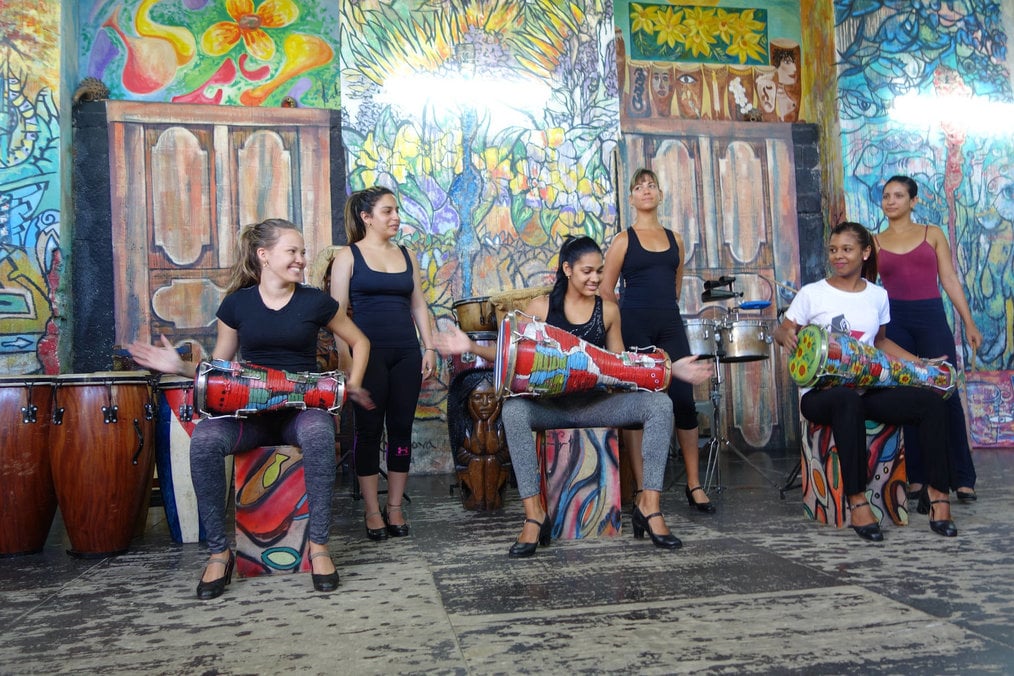The photograph depicts six young women, likely in their late 20s or 30s, positioned against a vibrant mural background that's adorned with bright and colorful flowers, including daffodils. Three of the women are seated on a colorful block, each holding vibrant bongo or congo drums on their laps. The woman on the left is wearing a tight black shirt, has blonde hair pulled back, and is accessorized with earrings. In the center, a woman with long, dark hair also pulled back and earrings is smiling, wearing a black tank top, gray pants, and black high-heeled shoes. Next to her, an African American woman in a white short-sleeved shirt gazes towards the center woman. All of them have ponytails and exude joyous expressions. In front of them lies a brown and beige carpet, while standing behind them are three other women dressed in coordinated attire—tight tank tops and yoga pants with dance shoes—likely preparing to dance. Also noticeable in the background are additional congo drums, an acorn-headed statue, and a large set of wooden bungo drums, adding to the festive, perhaps performance-focused atmosphere.